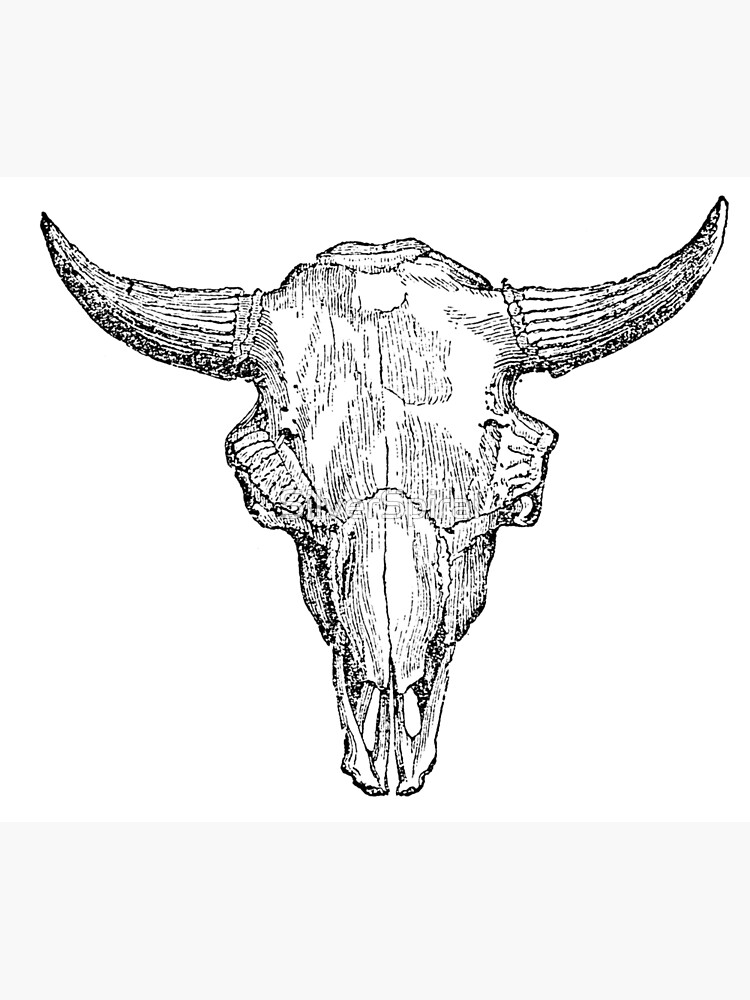This detailed black and white illustration depicts a cow skull, characterized by an intricate arrangement of black lines. The artwork shows the skull head-on, giving the impression it might be hanging on a wall or viewed from above. The skull's right horn is slightly longer than the left, with both horns depicted in darker, more substantial lines compared to the partially shaded forehead area. The eye sockets, mouth cavity, and teeth are rendered with varying line densities, providing a clear sense of the shading and contours. Although minimalistic and somewhat vintage in style, the precise dashed lines give it a contemporary New Americana feel, suggesting the piece could belong to any time period. A subtle, hard-to-distinguish silver ring sits on the front of the skull, adding a touch of modernity to this otherwise timeless sketch.